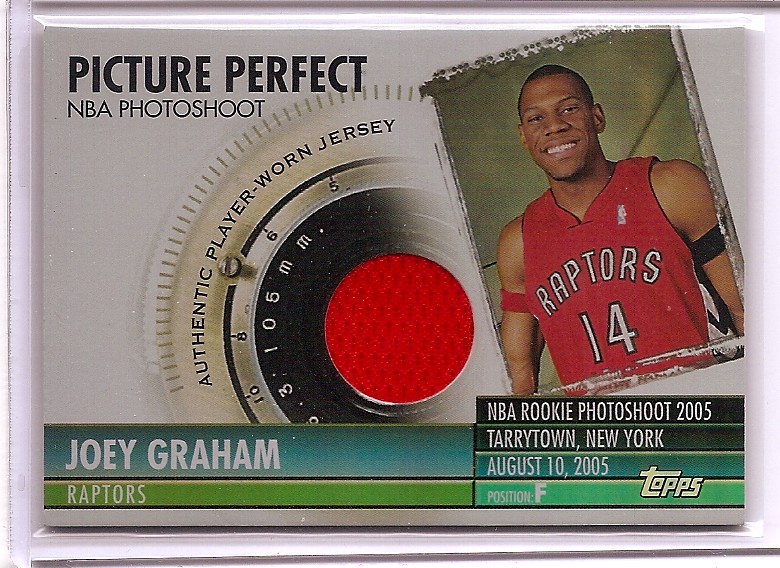This horizontal rectangular image is a Topps basketball card featuring a player from the Raptors. The upper right section showcases a tilted picture of Joey Graham, a black man sporting the Raptors jersey, which has the word "Raptors" in white letters with a black border above the number 14. He wears a black armband on one arm and a red armband on the other. In the top left corner, the card reads "Picture Perfect NBA Photo Shoot" with a dial-like image and a red button in the center, labeled "Authentic Player Worn Jersey." Along the bottom left, it states the player's name, "Joey Graham," and "Raptors." Below the picture, it's inscribed, "NBA Rookie Photo Shoot 2005, Tarrytown, New York, August 10, 2005." The overall card colors include white, off-white, black, tan, red, blue, green, and turquoise. The text "Topps" is also mentioned at the bottom.